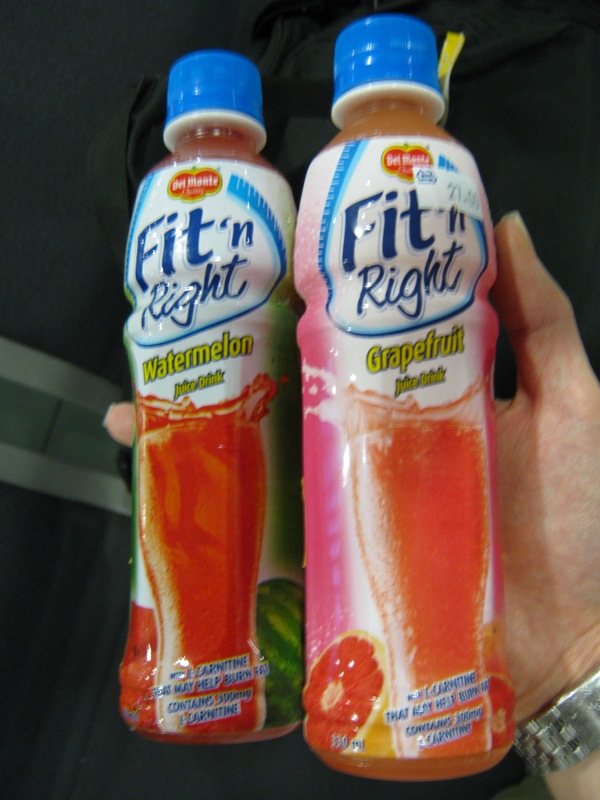In a vertically rectangular image, a deeply dark green background occupies the lower right corner. A right hand extends out at an angle towards the center, palm facing up, with the thumb partially visible but not the fingers. The hand is grasping two tall, slender, round drink bottles, each sealed with blue caps and branded with a white label featuring blue text that reads "Fit and Right". The bottles differ in flavor: the left bottle, labeled "Watermelon Juice Drink" in yellow text, displays a dark red liquid that appears to be splashing out of a curved, tall glass depicted further down the bottle. The right bottle, labeled "Grapefruit Juice Drink" in the same yellow text, portrays a dark pinkish-orange liquid similarly splashing out of its accompanying glass. The intricate details capture the vibrant, refreshing essence of the beverages.